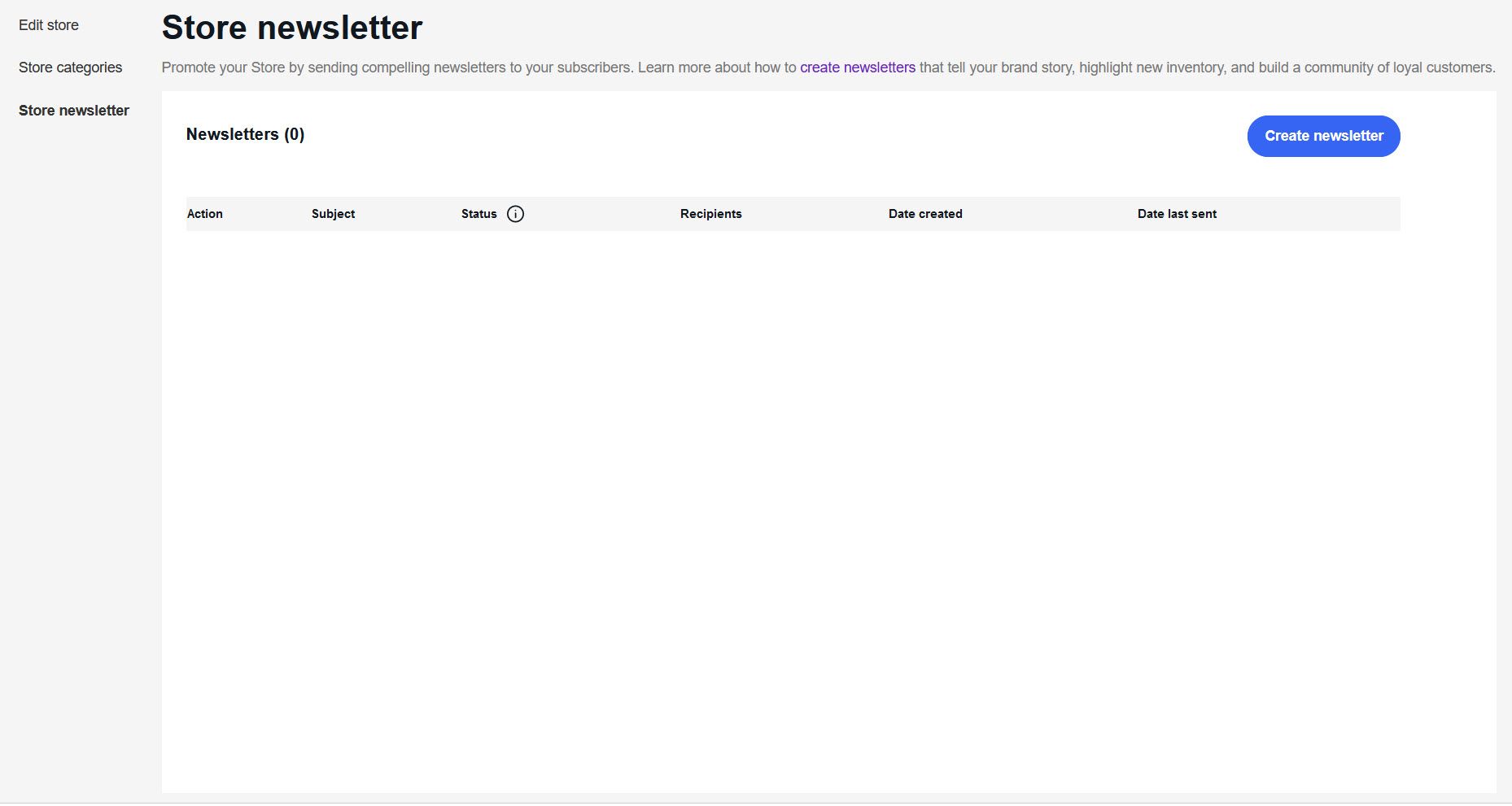The image depicts a webpage designed to support small mail order businesses in taking orders over the internet and keeping customers informed through newsletters. At the top left of the page, a title reads "Store Newsletter." Below the title, a gray sidebar facilitates navigation through three sections: "Edit Store," "Store Categories," and the currently displayed "Store Newsletter."

In the main content area, set against a white background, instructional text invites users to promote their store by sending compelling newsletters to subscribers. It encourages learning more about newsletter creation, with a link to "Create newsletters" explaining how to tell your brand story, highlight new inventory, and build a community of loyal customers. This introductory section is highlighted with a gray background.

The main white section of the page is relatively empty, showing no newsletters created yet, as indicated by "Newsletters (0)." On the far right, a prominent blue button with white text labeled "Create Newsletter" is visible. Below this, an empty table is prepared to list historical newsletters with columns for "Action," "Subject," "Status," "Recipients," "Date Created," and "Date Last Sent."